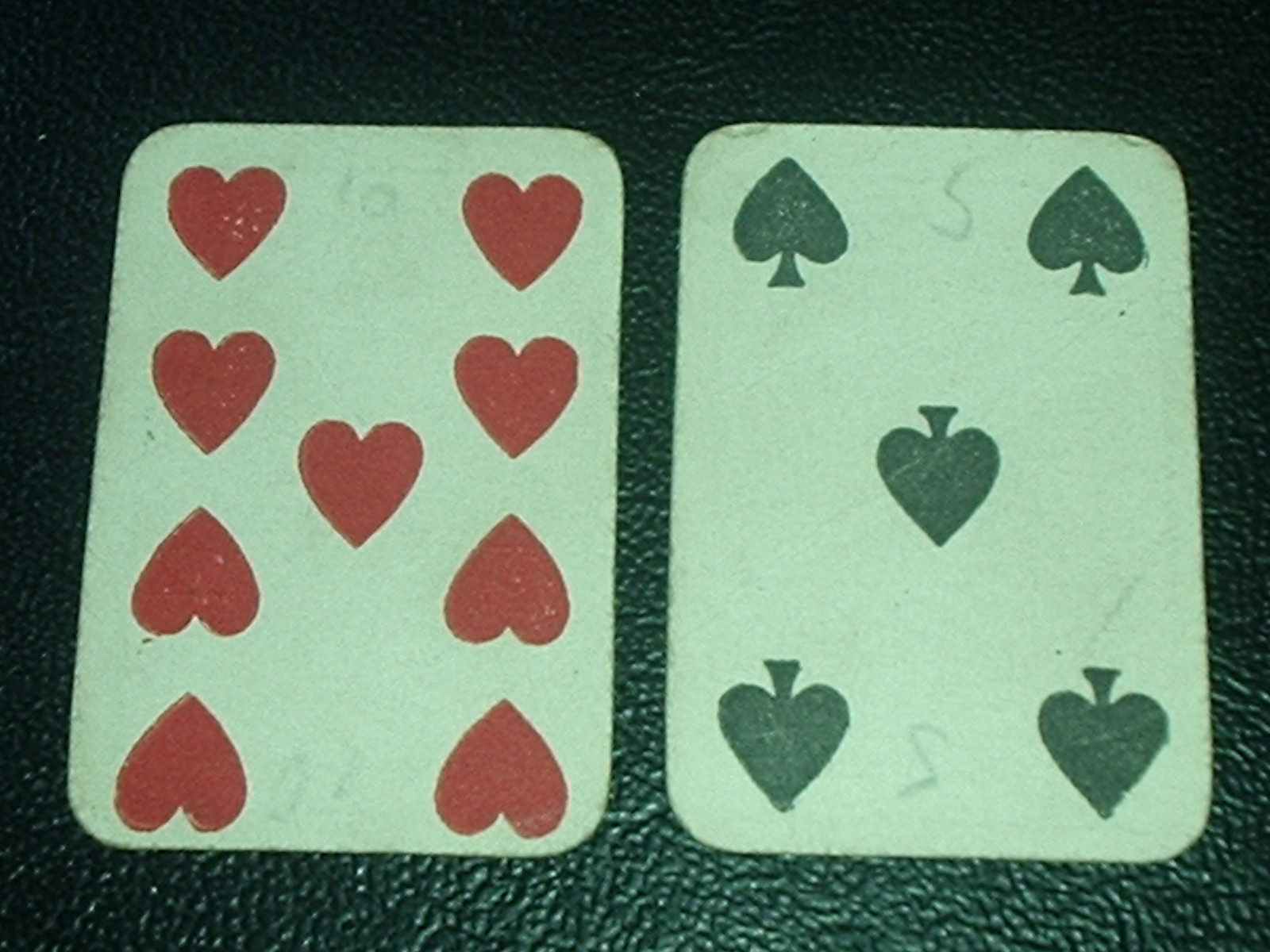In the image, two playing cards are positioned side by side, both face up, on a black surface with a texture reminiscent of leather. The worn nine of hearts is on the left, displaying visible dirt marks and signs of wear. Interestingly, at the top center of the nine of hearts, there's a penciled scribble that appears to say "ten." On the right is the five of clubs, equally worn and marked, with "five" scribbled at the top center in pencil. The bottom of both cards features reversed numbers: "01" on the nine of hearts and a reversed "5" that resembles an 'S' on the five of clubs. The cards, separated by a small gap, are identical in size, emphasizing their shared history of use and wear.